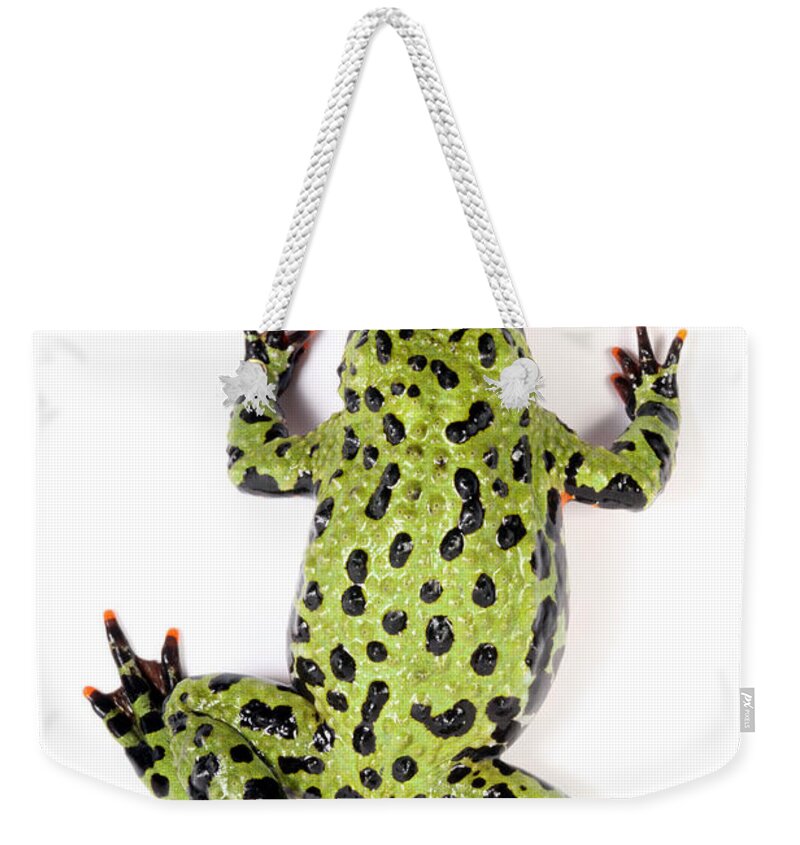This image showcases a unique handbag with a white background, featuring a green frog as its central design. The handbag is predominantly white, and the frog depicted on it appears photographic rather than illustrated. The frog is pickle green with black polka dots and orange-tipped toes. Its texture shows warts, giving it a lifelike appearance. The frog’s torso, part of the head, most of its two front legs, and one back leg are visible, but the full head is not. The bag’s handle is a silver metal chain, attached at either side of the frog’s head and arm, resembling washers or grommets. This professional image, likely intended for advertising, accentuates the color scheme of white, silver, green, black, and orange.